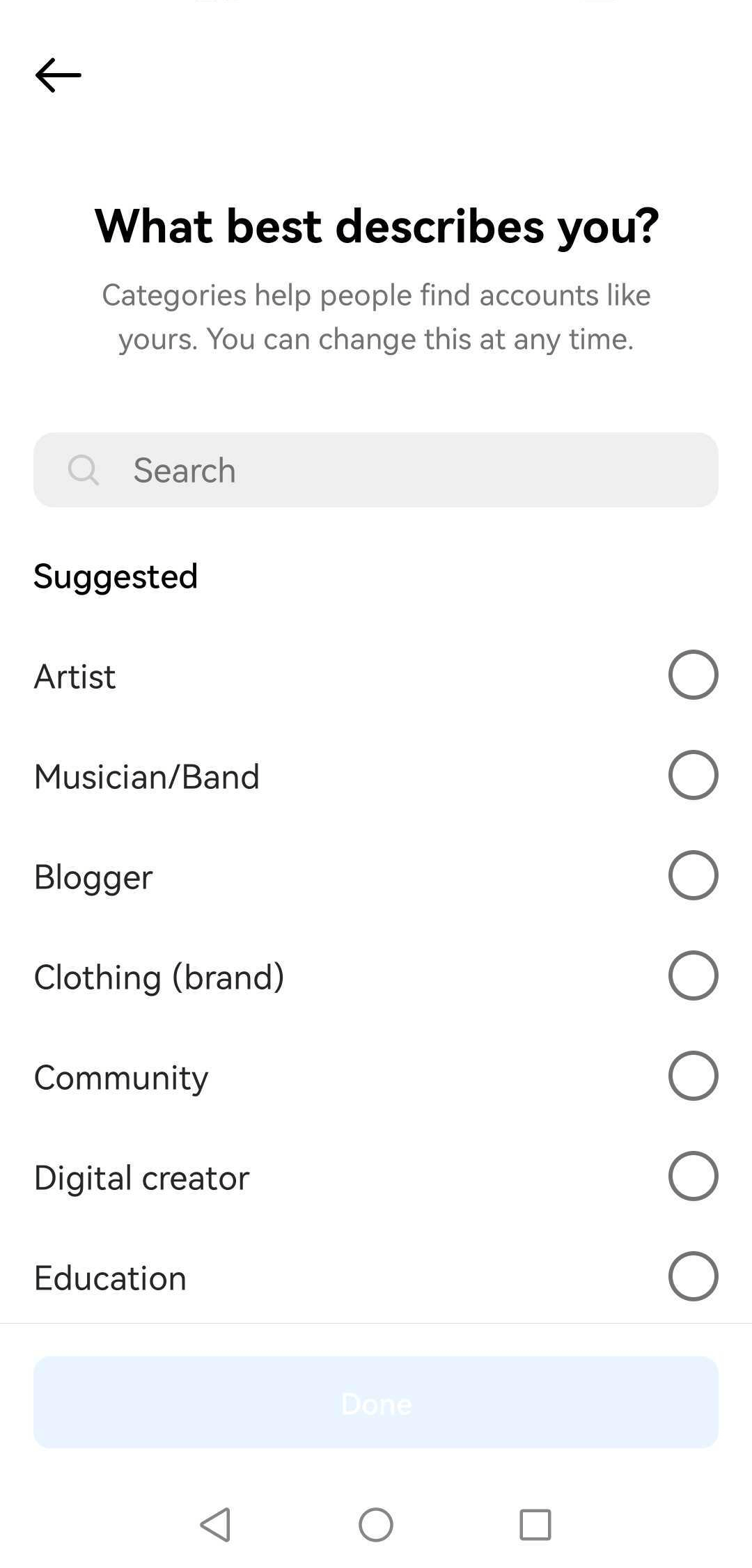This is a detailed caption for an image:

The screenshot captures a web page interface from a mobile device, as indicated by the standard cell phone icons at the bottom of the screen, including a triangle arrow button pointing left, a circle button in the center, and a square button on the right. 

At the top, in prominent bold, black letters, the page poses the question, "What best describes you?" Beneath this, a subheading in black letters states, "Categories help people find accounts like yours. You can change this at any time," suggesting this is part of a user profile setup or customization process.

Below the text, a gray horizontal rectangle features a search bar with a small magnifying glass icon on the left, offering a search function. 

Underneath the search bar, the section titled "Suggested" provides seven selectable categories with circles on the right-hand side, all of which are currently unmarked. The categories listed are: 
1. Artist
2. Musician/Band
3. Blogger
4. Clothing (Brand)
5. Community
6. Digital Creator
7. Education